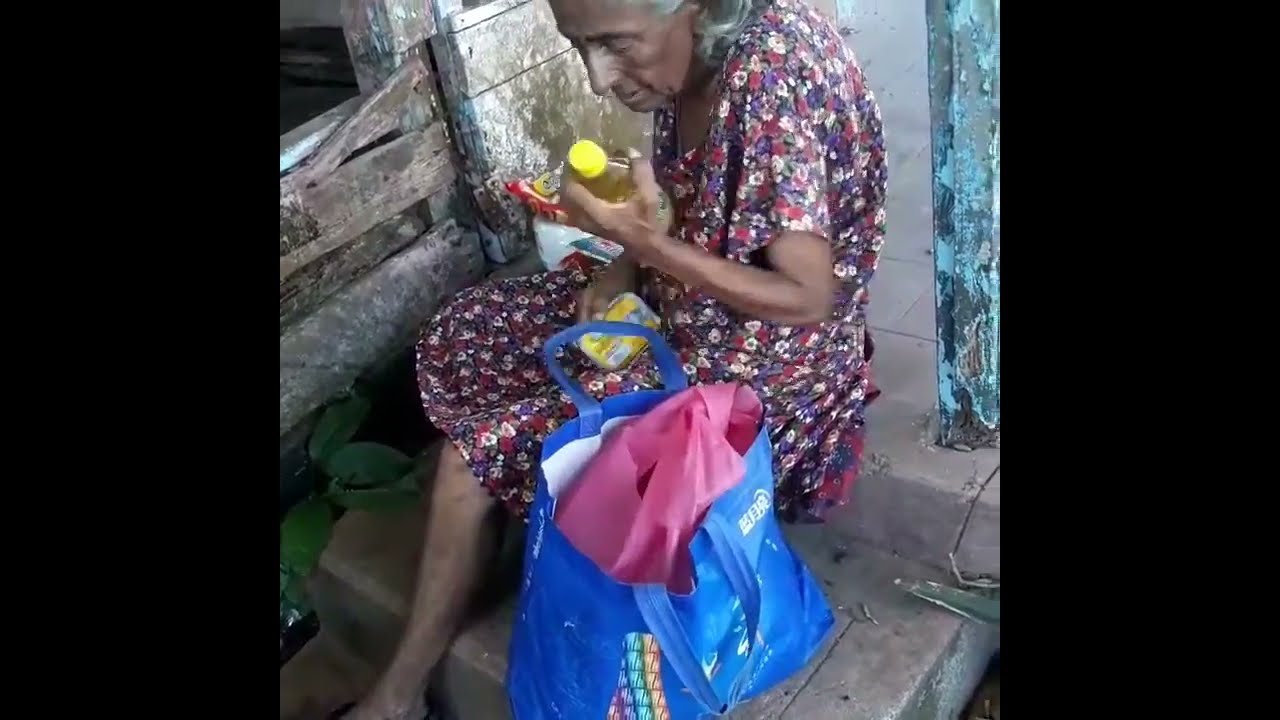In the photograph, an elderly woman with light brown skin and gray hair sits centrally on a concrete staircase, possibly in front of a house or an old dilapidated wooden structure. She is outdoors during daylight, suggesting a location that could be in a third-world country. Flanking the image are black vertical lines framing the border. The woman wears a multicolored, short-sleeve floral dress paired with flip-flops. To her right stands a greenish metal pole, while beside her rests a large blue tote bag containing a pink bag inside it. She holds various grocery items in her hands, including what appears to be a bottle and potentially a square metal box, possibly sardines. The background reveals structures in poor condition, and the overall scene is richly colored with hues of tan, green, white, blue, pink, yellow, light blue, and brown. The woman's posture and surroundings convey a sense of weariness and the passage of time.